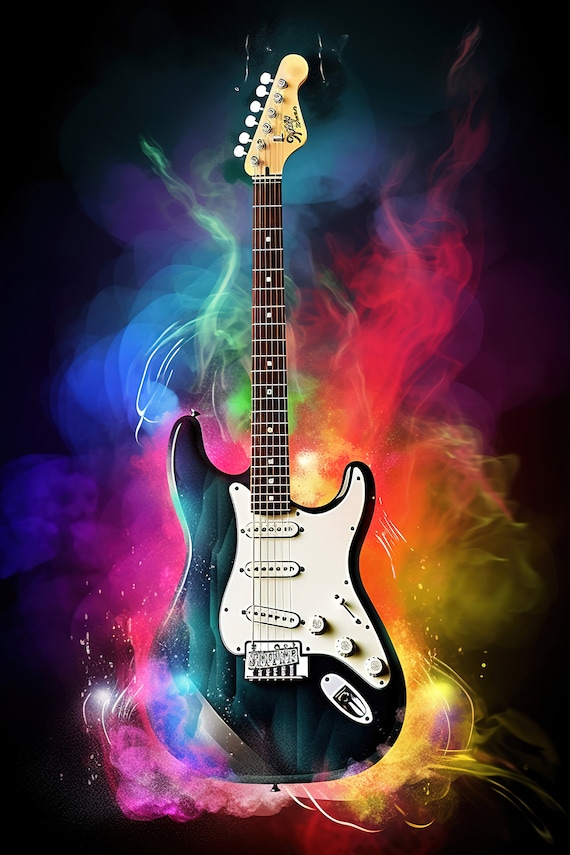The image is a stylized artwork featuring a traditionally shaped electric guitar, set against a black background. The guitar is positioned upright, with the pointed end of the neck at the top center and the rounded body at the bottom center of the image. The body of the guitar is a shiny, turquoise gem-like color, with a light brown wooden neck featuring multiple grey strings. The faceplate is white and adorned with intricate details such as three knobs with black notches and a sliding black knob. There is a silver teardrop shape on the body, likely for plugging in the guitar. Surrounding the guitar is a vibrant, smoky aura in a spectrum of neon colors—red, orange, yellow, green, blue, indigo, and violet, along with shades of pink and white—adding a dynamic, almost ethereal quality to the scene. The smoke appears to embrace the guitar from all sides, except for the very top, enhancing the overall vivid and colorful composition.